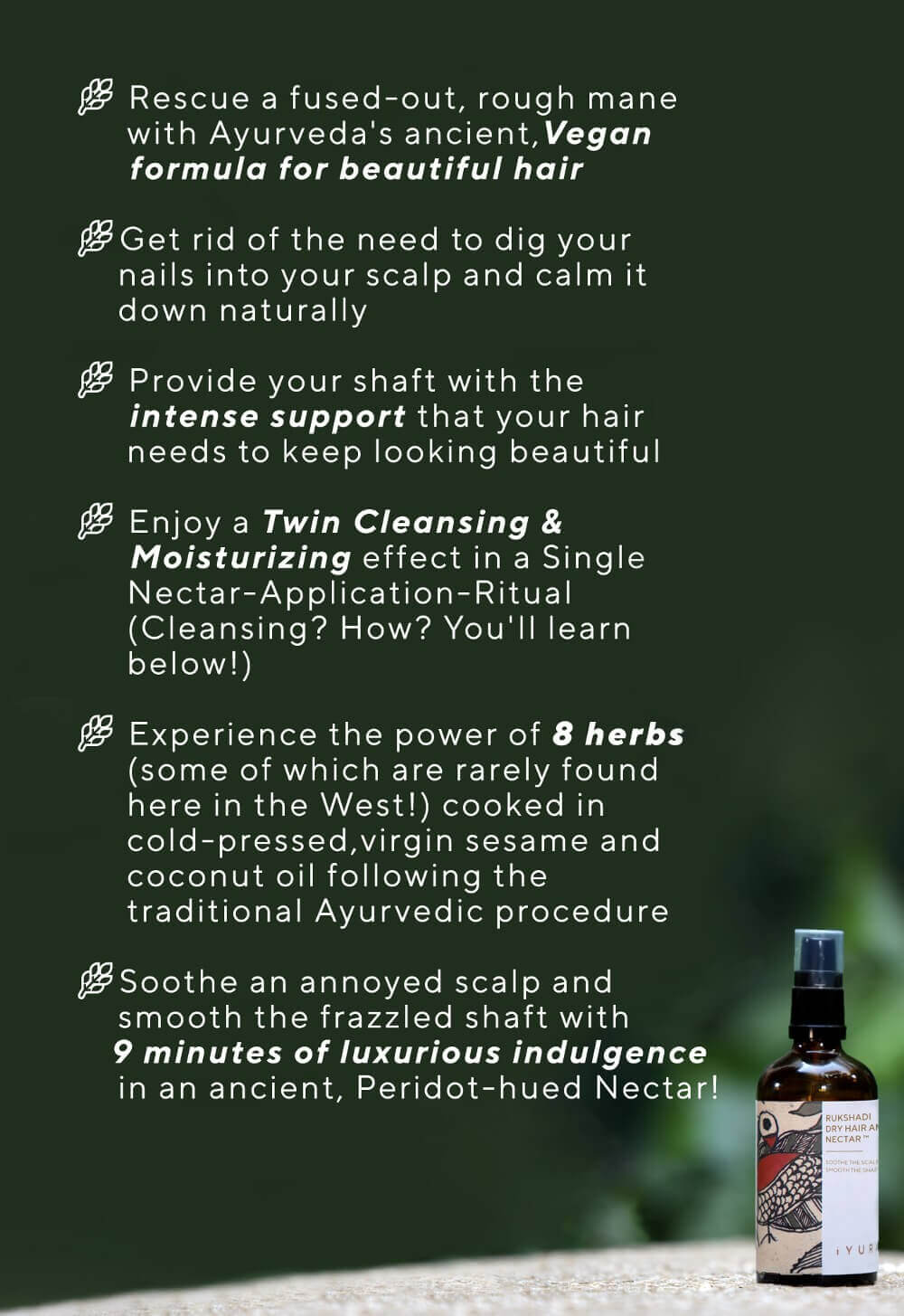This advertisement showcases an Ayurvedic hair care formula designed to rescue a frizzy and rough mane using an ancient, vegan concoction. The main text, divided into six sections, emphasizes its benefits and unique composition. It highlights calming the scalp naturally, providing intense support to hair shafts, and offering a dual cleansing and moisturizing ritual with a single application of peridot-hued nectar. The formula includes eight rare herbs, prepared in cold-pressed virgin sesame and coconut oils, following traditional Ayurvedic procedures. The ad promises nine minutes of luxurious indulgence to soothe the scalp and smooth frazzled hair. Accompanying the text is an image of the product—a small brown glass bottle with a plastic cap featuring unclarified imagery in black, white, and red, labeled "Rukshadi, dry hair and nectar." The backdrop is a rich, dark green, with white text creating a stark contrast. On the bottom, the letters "IYUR" hint at the product's name.